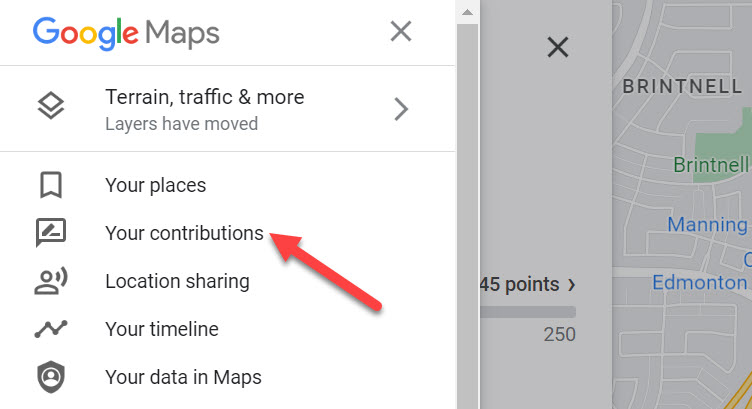The image is a zoomed-in screenshot of the Google Maps interface, divided into two primary sections. On the left side, the title "Google Maps" is prominently displayed at the top. Directly to its right is an "X" button for exiting the page. Just below the title, there are options labeled "Terrain," "Traffic," and "More," accompanied by a button that opens an additional menu. Further down, users can see five different options: "Your Places," "Your Contributions," "Location Sharing," "Your Timeline," and "Your Data in Maps," each with a corresponding icon to the left.

Adjacent to the left section, the right side of the image features a partially visible map, showcasing the locations of various cities. An "X" button is situated in the upper left corner of this map segment, allowing users to close the map view. 

On the left side, a large red arrow points diagonally towards the "Your Contributions" option, creating a subtle shadow effect. The background of the entire screenshot is a clean white, emphasizing the interface elements without any additional distractions.